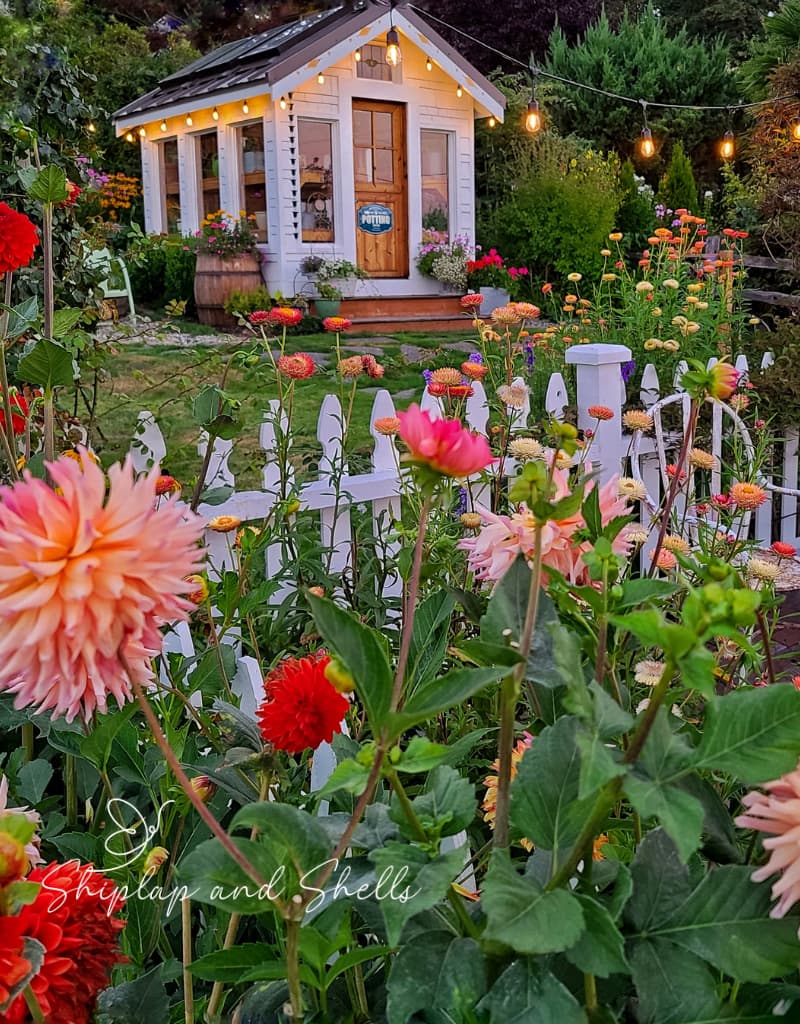A picturesque garden with a vibrant variety of flowers, predominantly dahlias in shades of pink, yellow, and white, blooms abundantly in the foreground, enclosed by a charming white picket fence. The serene setting features a quaint white and gray shed, styled like a tiny house, with shiplap siding detailed in the text "shiplap and shells." The shed stands amidst lush greenery, ornamental bushes, and a barrel brimming with plants. Bright white string lights adorably adorn the roof and trail off to a nearby tree, illuminating a cozy sitting area with a solitary chair. The shed’s dark gray roof and brown front door provide a striking contrast against the garden’s colorful and fragrant palette, creating an inviting and tranquil atmosphere.